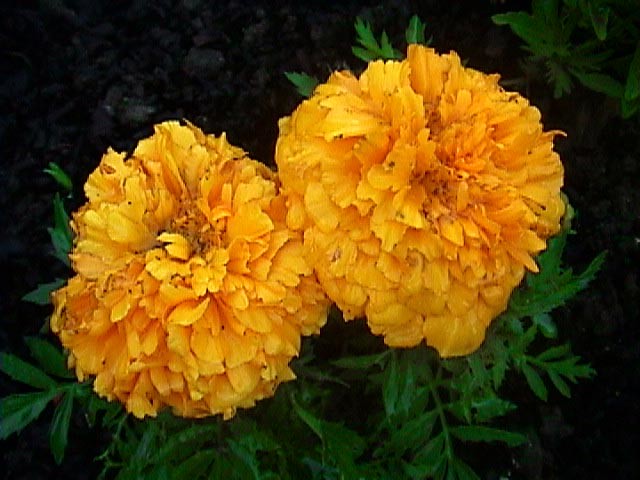This image captures two vibrant marigold flowers in full bloom, showcasing their intricate clusters of orange-yellow petals with a slightly flaky texture. Both flowers are rounded and sit side-by-side, with the one on the right positioned slightly higher than the one on the left. The background features green leaves branching off their stems, providing a lush contrast to the blooms. The scene is set against a somewhat dark background, with more leaves visible in the upper right corner and a hint of soil and possibly rocks in the back left. The overall setting emphasizes the rich, colorful beauty of the flowers amidst their natural garden environment.